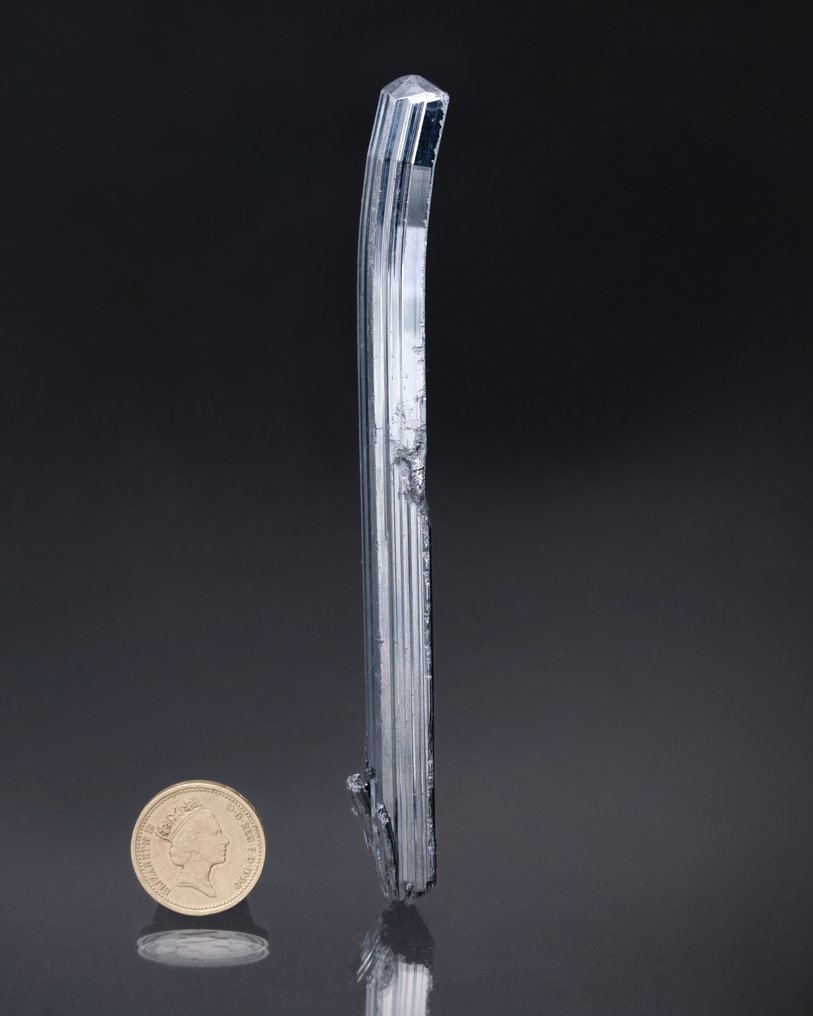The image depicts a highly reflective silver metal object and a coin, both displayed on a glossy, black glass-like surface, creating a clear reflection. The metal object, positioned slightly to the right, is long, thin, and shiny with a curve and a protrusion near its lower end, and it appears deformed or bent towards the middle. On the left, the coin is a British pound, recognizable by the gold color and the image of Queen Elizabeth on its face. The background is entirely grey, enhancing the reflective quality and focus on the items displayed.